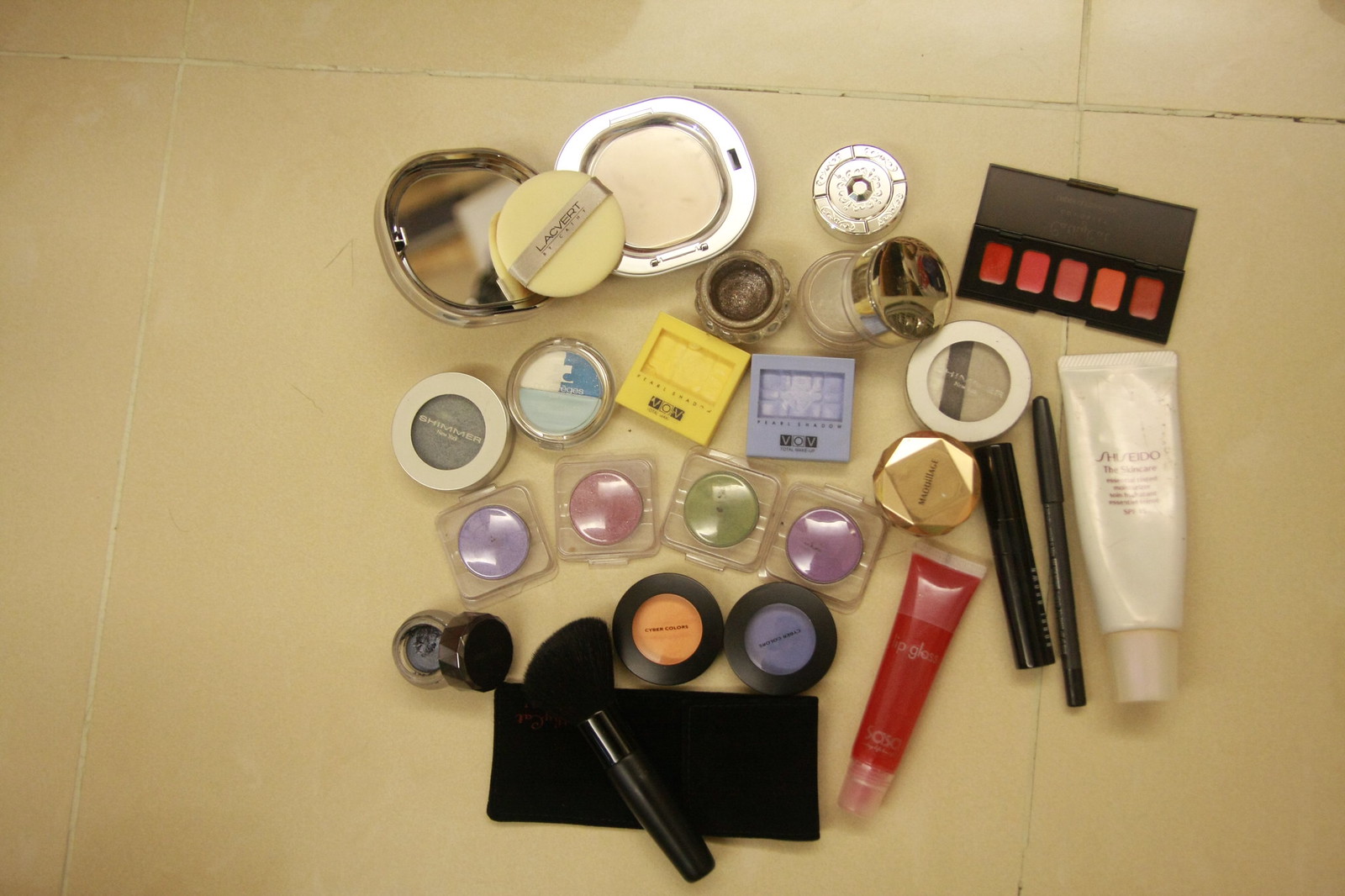This overhead image captures a collection of various makeup products scattered on a beige ceramic tile floor, revealing grout lines that appear aged and slightly dirty. Among the assortment:

- **Central Compact**: An open compact displaying a small, yellow circular powder puff.
- **Assorted Small Jars**: 
  - A small glass jar with a silver lid.
  - A plain small silver jar.
  - An open glass jar containing a bronze-hued cream product, likely cream eyeshadow.
- **Right Side Ensemble**: 
  - An open black palette featuring five warm pink shades, potentially a lip palette.
  - Beneath the palette, a white tube labeled with the Shiseido brand.
  - Adjacent items include a black eyeliner pencil, a black tube of mascara, and a clear tube filled with pink lip gloss.
- **Additional Items**: 
  - A gold-colored item.
  - Several eyeshadows in vibrant colors: purple, green, pink, light purple, orange, and blue.
  - A pot of gel eyeliner and a makeup brush.

The image offers a detailed snapshot of the diverse makeup collection against the contrasting backdrop of the tiled floor.